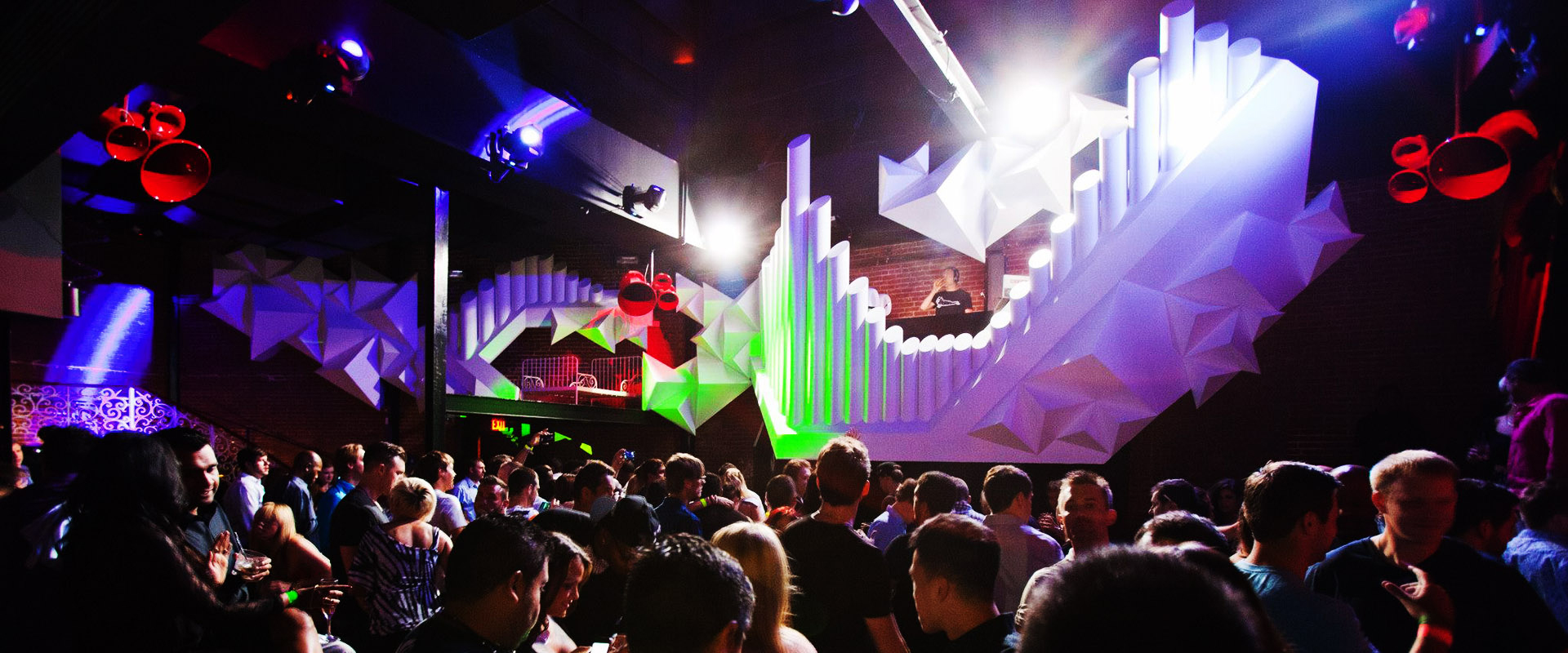In this indoor photograph, we observe a bustling concert venue or nightclub, heavily veiled in darkness. The lower third of the image reveals a packed crowd, partially cast in shadows. Above them, a brightly lit stage commands attention. A central figure, likely a DJ, is positioned towards the back of the stage, distinguishable by the headphones they are wearing. 

The stage is adorned with various artistic decorations, prominently featuring a large white structure resembling a series of vertical bars, akin to volume indicators on a music editing software, extending and transforming into geometric shapes. This intricate 3D-printed prop adds a unique and captivating element to the venue's ambiance. Surrounding the stage are red alarm-like horns in groups of three, along with clusters of LEDs that bathe the scene in vibrant hues of green, pink, and blue, adding further color to the already dynamic environment. A powerful white light from the ceiling illuminates the central area of the stage, enhancing the overall effect and making the venue both visually stimulating and immersive.